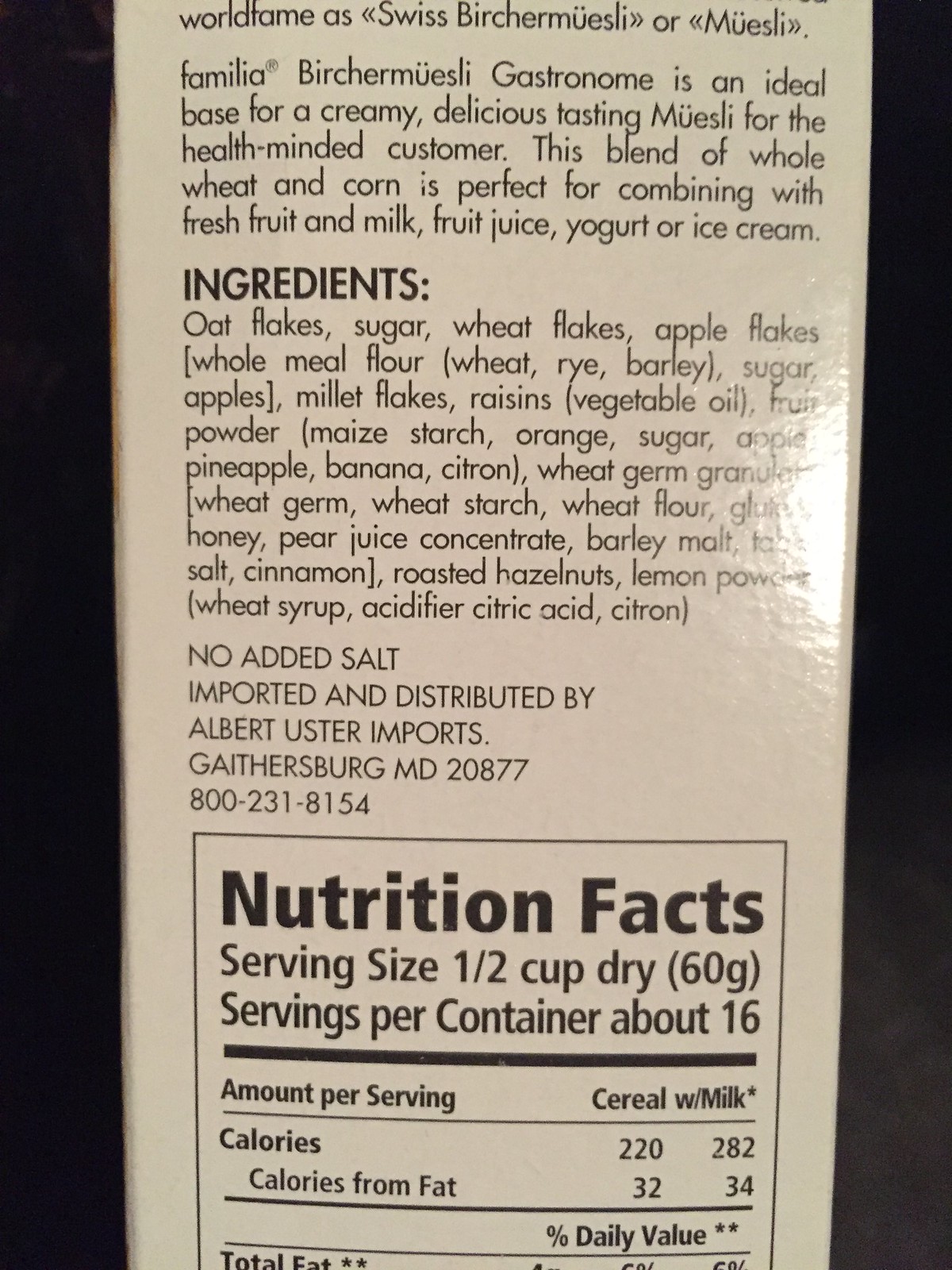The image is a color photograph of the side of a muesli cereal box with a black background and a slightly beige-tinted cream label. At the top, the label includes text such as "World Fam" and "Familia" in black lettering, although it is not entirely visible. Below this, within a squared-off area, the nutritional facts are partially shown, detailing serving sizes and calories per serving. 

A bright light is shining on the right edge of the label, highlighting the detailed list of ingredients including oat flakes, sugar, wheat flakes, apple flakes, whole meal flour, rye, barley, millet flakes, raisins, vegetable oil, pineapple, banana, citron, pear juice concentrate, wheat germ, wheat starch, wheat flour, gluten, honey, malt, salt, cinnamon, roasted hazelnuts, lemon, wheat syrup, and acid citron. Bold letters emphasize items like "no added salt." 

Additionally, the product is imported and distributed by Albert Uster Imports from Gaithersburg, Maryland, with a specific address and phone number. The nutrition facts specify a serving size of half a cup dry (60 grams), with about 16 servings per container, noting both calories per serving (220 with milk), and calories from fat (32).  The image captures the comprehensive and detailed product information despite being cut off at the bottom.